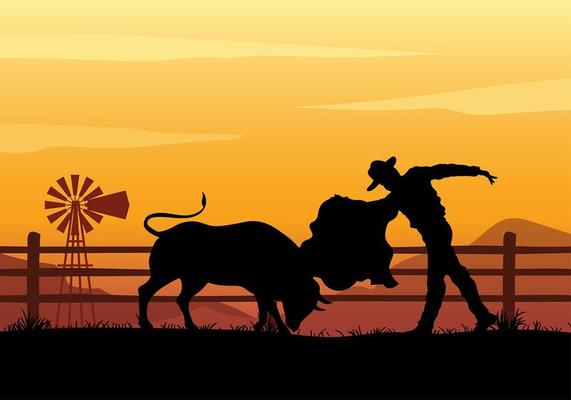This pixel art image, about four inches wide and three inches high, vividly depicts a dramatic bullfight scene. The silhouetted black figures of a bull and a man dominate the composition: the bull, on the left, charges with its head lowered, tail raised; the man, on the right, leans forward, bracing himself on his left leg, and waves a vibrant cape, adorned with a cowboy hat. A light brown wooden fence, composed of three horizontal bars supported by evenly spaced posts, extends across the middle ground. The silhouette of the ground features thin black grass shoots sprouting upwards. Behind the fence, the background showcases a reddish-brown windmill silhouette and a range of orange-brown mountains. The sky above is painted in yellow hues, suggesting a serene sunset, with paler yellow clouds streaking horizontally across it. This detailed scene may appear either as a traditional painting or a computer-generated image.